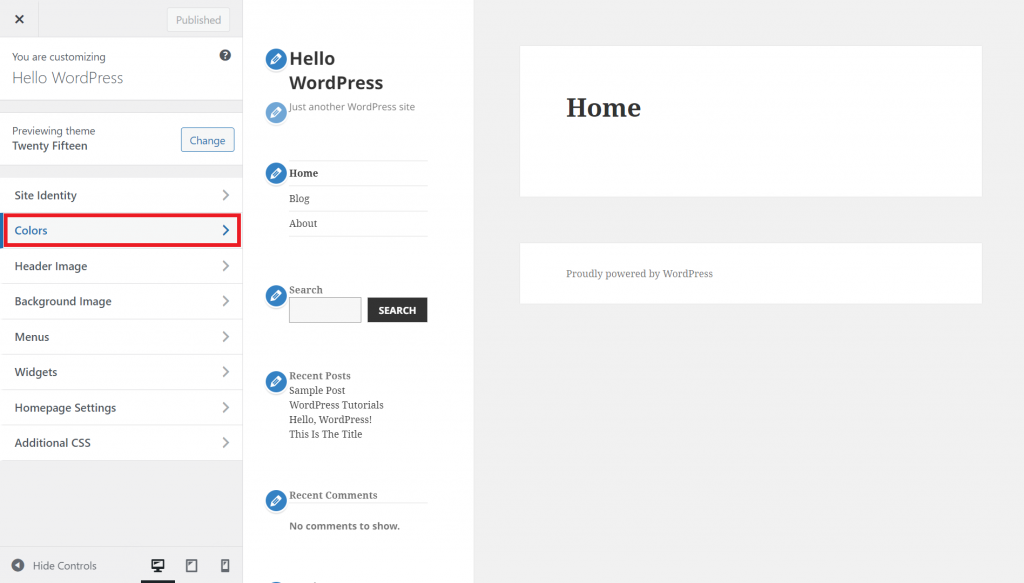**Image Caption:**

This image showcases a website interface divided into three distinct sections. 

- **Left Section (Gray Column):** This long, vertical rectangle extends down from the top approximately a quarter of the way across the screen. At the top inch of this gray section, there is a black "X" in the corner. Below this, towards the right, is a lighter gray tab labeled "Published.” Underneath this tab, a white section reads "You are customizing." Below this, in gray text, it says "WordPress" with a gray border. Further down, the white section reads "Previewing theme 2015," with a blue tab to the right labeled "Change" in dark blue. The gray section then becomes white, except for the bottom two inches, which feature various settings: "Site Identity," "Colors" (highlighted in blue with a red rectangle around it), "Header Image," "Background Image," "Menus," "Widgets," "Homepage Settings," and "Additional CSS." At the bottom left, a gray border contains "Hide Controls.” In the bottom right corner, there are two picture icons and a monitor icon.

- **Middle Section (White Column):** This section is completely white and occupies another quarter of the screen's width.

- **Right Section (Gray Background):** The top of this section has a large gray rectangle with the word "Home" centered on the left side. Below this, in black text, it says "Hello World Press," next to which is a blue circle featuring a white pencil outline. This section continues down with five additional blue circles with white pencil outlines, each containing various information. At the very bottom, it reads "Proudly powered by WordPress."

Together, these sections detail the site's customization interface, providing a visual guide to the layout and various control panels available for the user.